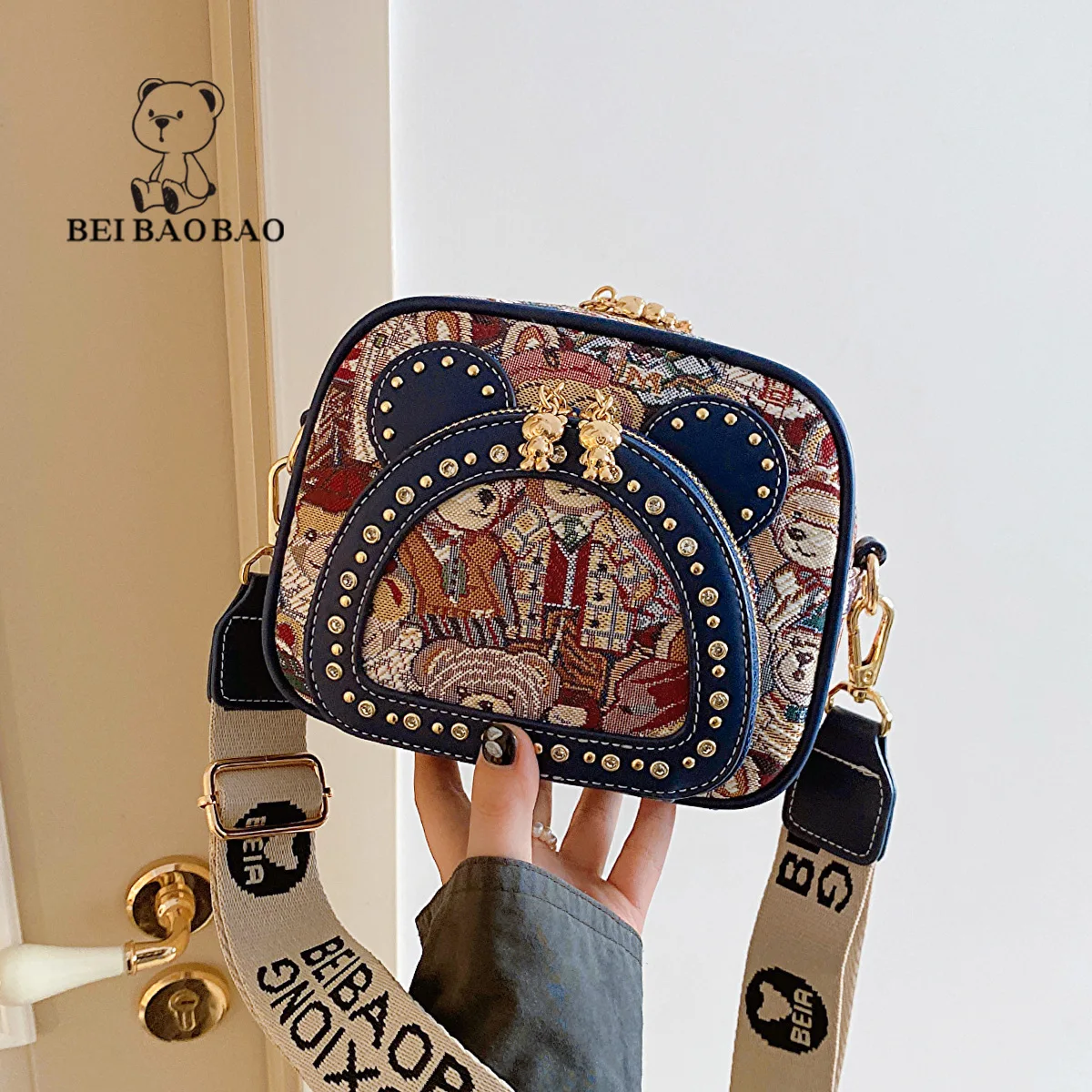This is a detailed product photo of a delicately embroidered handbag with a teddy bear aesthetic. The handbag is woven with fabric that resembles a decorative throw blanket, featuring a colorful tapestry of teddy bears dressed in human clothing. It has a lunchbox-like, square shape with a semi-circle front pocket adorned with little bear ears on the sides. The bear figures are also present on the zipper pulls. The purse has a woven strap, predominantly white, inscribed with the brand name "Bay Bow Bow." 

The purse itself is held by a Caucasian hand with black and gold leaf-decorated fingernails, only the thumb visible with four fingers behind it. The purse is directly facing the camera, framed against a white wall and an off-white door with a gold and acrylic handle. The design features an oval shape with a blue border and a thick blue leather semi-circle. Additional semi-circles contour to form a bear's shape. There are seven visible teddy bears in human form on the intricate knitted surface. Text on the strap reads "BEIA," and a blue teddy bear drawing along with text "Bay Bow Bow" is present in the top left of the image.